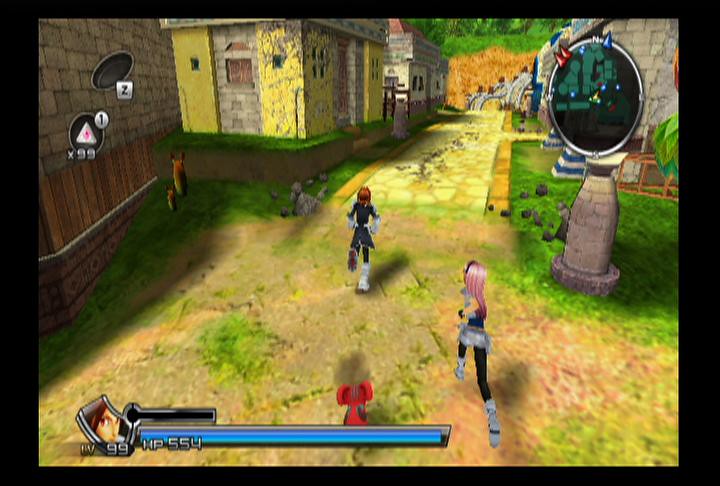The image is a detailed screenshot from a video game scene, featuring a variety of elements both within the game and on the screen interface. The game window is bordered by a wide black frame, which is thicker on the sides and narrower on the top and bottom. In the gameplay area, three characters are running towards a yellow brick road that leads to a series of buildings in the background. The path, reminiscent of the yellow brick road from classic tales, is edged in a stronger shade of yellow. Beyond the path, there's a bridge leading to gold-colored cornfields and distant vegetation, hinting at a rich, expansive landscape. On the left of the path stands a dilapidated yellow house with peeling paint, followed by a cream-colored house. Behind these structures is a stone wall resembling those found in castles, fenced off by wood and a red brick wall at the base.

In the game's interface, the bottom left corner displays a status bar containing a character's face inside a geometric shape, with a blue horizontal bar indicating HP, reading 554 HP. Next to this, "LV99" is clearly marked, denoting the character's level. On the top right corner, there's a map radar encased in a reflective gold border with compass points indicated (N, E, W, S). The map shows various geometric shapes in green, blue, and red, with a yellow triangle marking the player's position. Additionally, a black circle on the left side of the screen contains a white triangle and "X99" beneath it, along with a "Z" on the top part. The ground in the game scene features overgrown weeds and some grass, adding to the immersive environment.